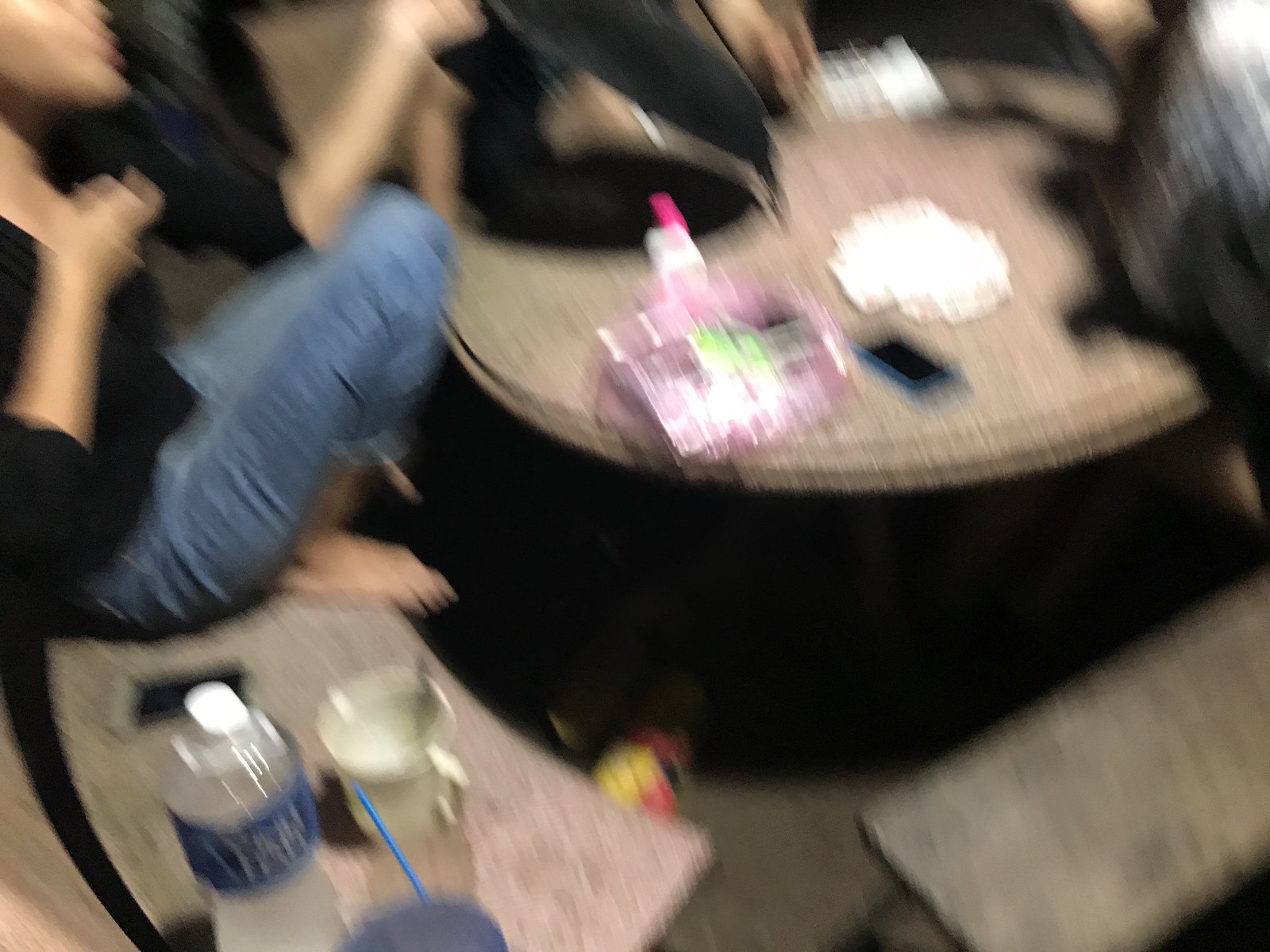This slightly rectangular, landscape-oriented photograph captures a group of people seated around a circular, light brown table. The image is notably blurry, but the woman most clearly visible is positioned in the upper left corner. She is dressed in a three-quarter sleeve black shirt paired with blue jeans. Adjacent to her, a bottle of water and a cell phone are noticeable on the table. Additionally, another cell phone and a black bag are present on the tabletop. Various other individuals are also seated around the table. Encircling the table is a bench of the same light brown hue, providing seating for the group.